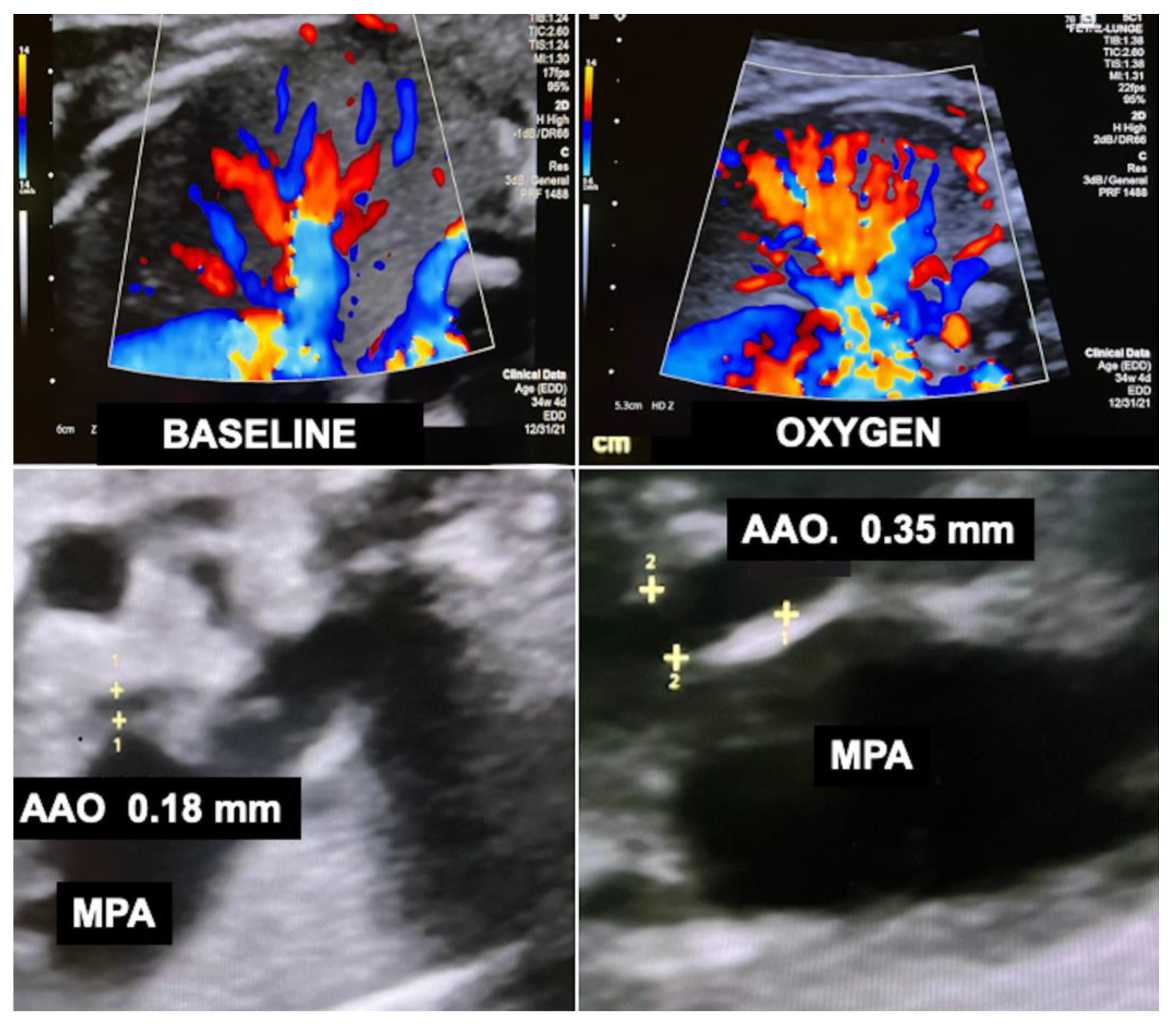This image is a detailed medical scan divided into four distinct sections, with the top two images in vibrant colors and the bottom two in black and white. The top left image is labeled "baseline" and features a colorful array of blues, reds, and oranges. Adjacent to it, the top right image, labeled "oxygen," displays an even more vivid spread of the same colors against a darker background. Both images appear to illustrate different stages or conditions, possibly related to oxygen levels in tissue or fluids, given the color variations.

The bottom left section showcases a grayscale image labeled "AAO 0.18 mm MPA," featuring various markers and annotations. Similarly, the bottom right section, labeled "AAO 0.35 mm MPA," presents another grayscale image with several indicators, including a distinct yellow plus sign, suggesting specific points of interest or measurement. Together, these images provide a comprehensive view, potentially highlighting changes in a medical condition over different parameters.